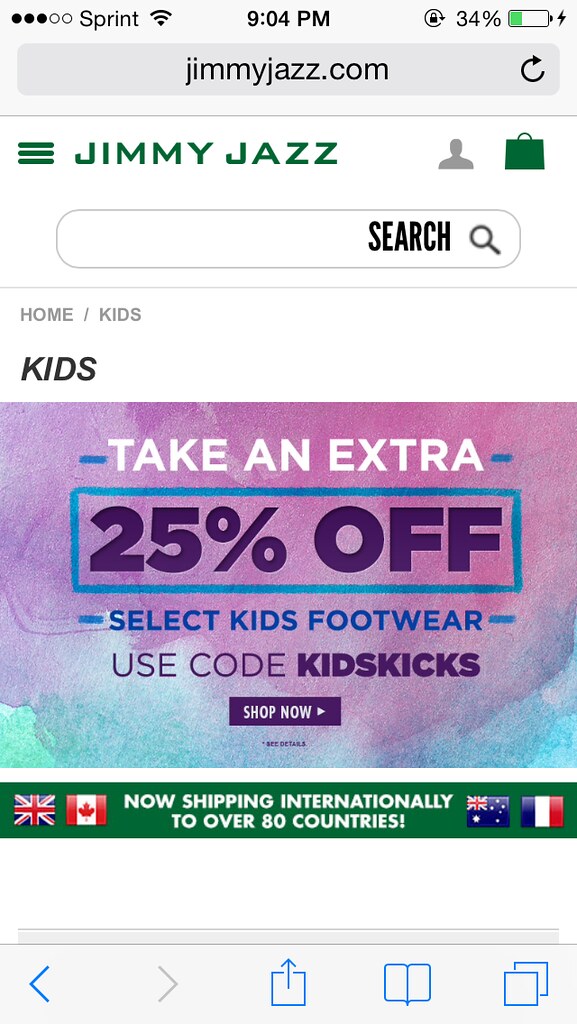The image is a detailed mobile screenshot captured at 9:04 p.m. on a phone using Sprint, with a 34% battery level remaining. The phone's status bar shows a connectivity symbol next to the word "Sprint" on the left. The time is displayed in the center, and a battery icon is in the top right. Below the status bar is a gray horizontal bar featuring the text "JimmyJazz.com" on the left, and a refresh symbol on the right.

The main content starts with a black menu bar on the left, and icons for an avatar and a suitcase on the right side of the gray bar. Below this, a search bar is outlined in gray with the text "SEARCH" and a magnifying glass icon on the right. Following this, a navigation bar shows "Home / Kids" in capital letters.

Prominently, an advertisement with a purple and blue gradient watercolor background is present. The ad contains the following text in white, dark purple, and blue sans-serif fonts: "TAKE AN EXTRA," followed by "25% OFF" within a blue-outlined rectangle. Below this, it reads "Select Kids Footwear" and then "Use Code KIDSKICKS" in bold. A white "Shop Now" button with a right-facing arrow is also visible. Underneath the ad, a thin green bar reads "Now shipping internationally to over 80 countries" in white text, flanked by flags of the UK, Canada, another flag with a blue field and white stars with a Union Jack in the corner, and the flag of France. Further below is the phone's function menu.